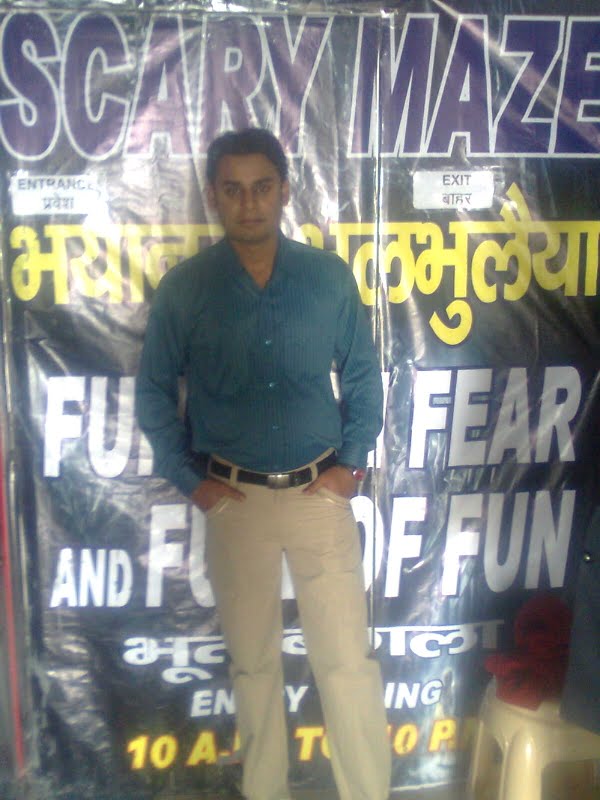This image features a well-dressed gentleman in his 30s or 40s with a short dark hairstyle and a tan complexion, possibly of Middle Eastern or South Asian descent. He is standing in front of a large billboard that promotes a "scary maze" attraction, emphasizing "fear and fun." The billboard includes text in both English and a South Asian language, possibly Thai or Hindi. The man is wearing a blue button-up shirt with stripes, beige khaki pants, and a black belt, with both hands casually placed in his pockets and his thumbs out. He also sports a watch with a red face on his left wrist and maintains a professional yet neutral posture, looking directly at the photographer. To his right, there's a small stool with some items on it. The location appears to be an entrance or exit for the maze attraction, likely situated in a South Asian region.